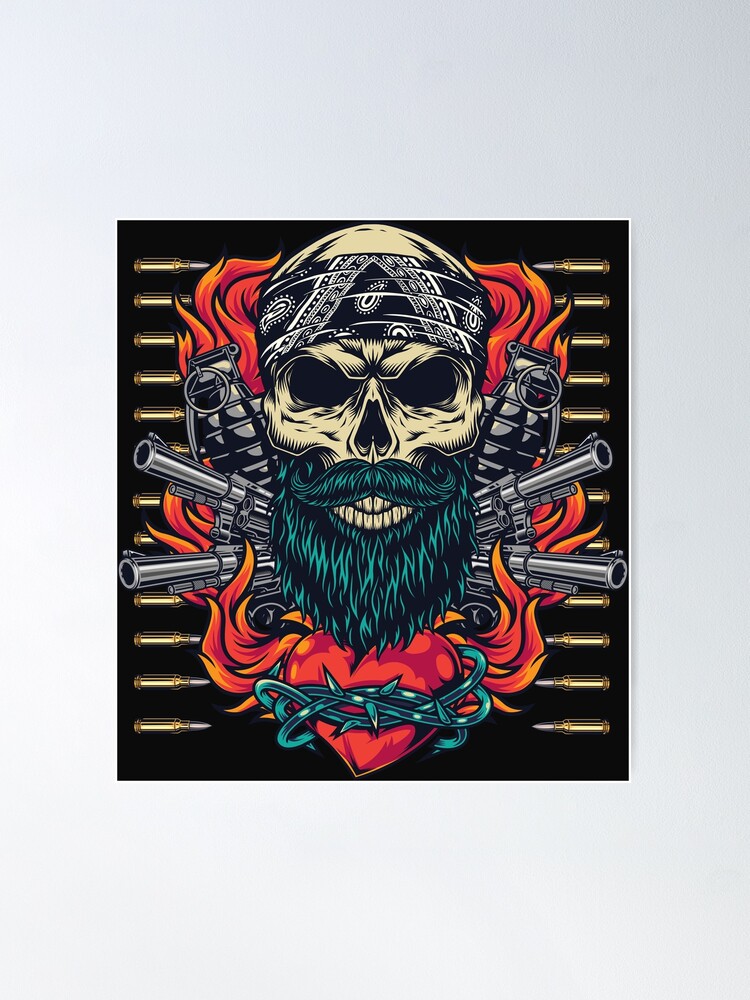This digital artwork features a stylized, off-white skeleton with a prominent teal-colored beard and mustache. Adorning its head is a black and white bandana, and its mouth is open, revealing prominently displayed teeth. Flames of reddish-orange fire erupt behind the skeleton, contrasting sharply with the solid black background. Positioned as if they are ears, two grenades flank the skull, while four gun barrels extend outward from the beard—two on each side—adding to the image's menacing tone. Below the beard rests a red heart, tightly wrapped in barbed wire, which also includes some orange circles for added detail. Surrounding the heart and framing the sides of the image are silver-tipped, gold-colored bullets, reminiscent of rifle ammunition. These bullets point inward toward the skeleton, which adds to the overall aggressive and violent aesthetic. The entire artwork is cartoony in style and bears a tattoo-like quality.